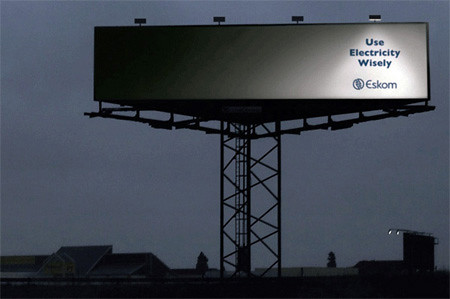In this grayscale nocturnal scene, a large illuminated billboard prominently stands on a stark black scaffolding framework. Placed high in the nighttime sky, the billboard features a succinct message on its right side, written in blue print: "Use Electricity Wisely." Beneath this advisory, the name "Eskom" is displayed, identifying the electricity company responsible for the message. Four lights are situated above the billboard, yet only one is activated, casting a focused beam over the crucial text, thereby emphasizing its importance. Below this elevated display, the tops of what appear to be homes or businesses are faintly visible, with only their roofs discernible in the dimly lit environment.